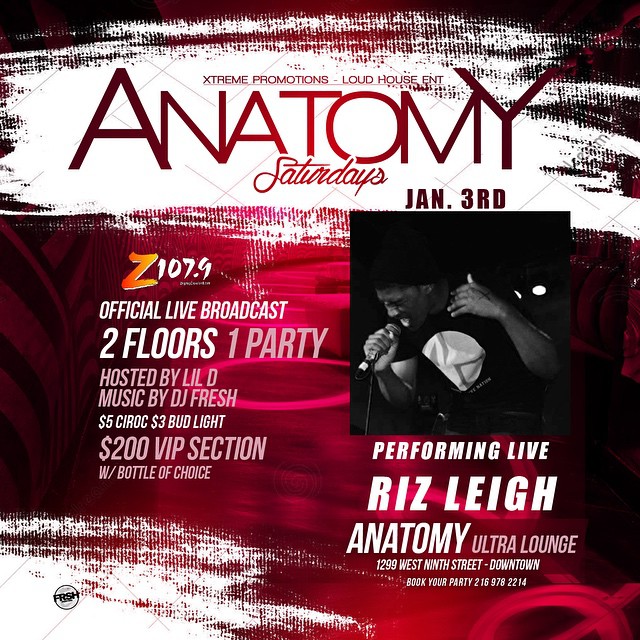This square image, likely a poster for an event, prominently features a dark and abstract background in shades of red and black. The striking design includes streaks of red, topped with a wide, prominently white streak where the word "ANATOMY" appears in large red capital letters. Above this, in very small print, are the words "XTREME Promotions - Loud House ENT." Below "ANATOMY," "Saturdays" is elegantly written in cursive. Underneath, bold black text highlights the event date: "Jan 3rd."

The right side of the poster displays a black and white image of a dark-skinned man wearing a black hat and t-shirt, singing into a microphone. Adjacent to this image are details of the event: "Performing Live Ree's Leigh," "Anatomy Ultra Lounge," and the address "1299 West 9th Street Downtown."

On the left side of the poster, additional information includes: "Z107.9 Official Live Broadcast," "Two Floors, One Party," "Hosted by Lil D," and "Music by DJ Fresh." Promotional offers such as "$5 Ciroc" and "$3 Bud Light," along with a "$200 VIP section with bottle of choice," are also noted.

The overall impression of the poster is dynamic and vivid, with elements blending into a visually engaging mix of dark tones, highlighted by the glowing pink, red, and white accents. The streaky paint lines and scribbles add an abstract artistic flair to the captivating design.